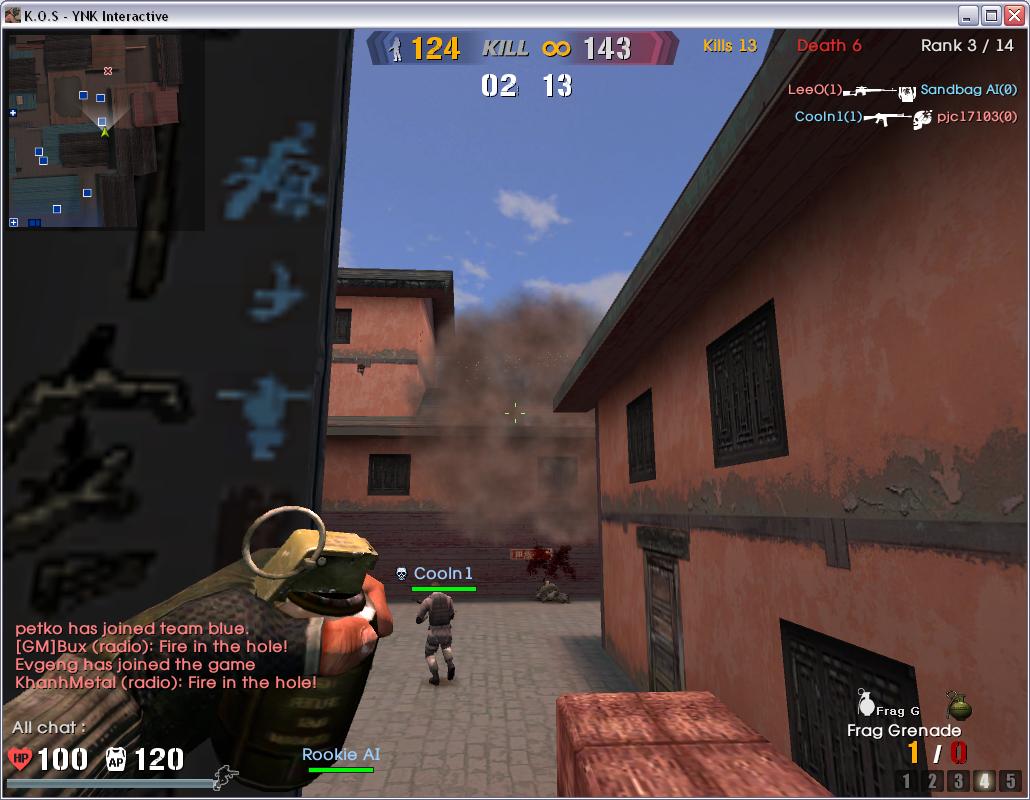The image depicts a video game screen featuring a character positioned in the lower center of the frame, facing away from the camera. The character is clad in brownish-gray attire. To the right of the character and in the background, there are several orange and dark-orange buildings. In the foreground, there is a large orange crate section, adding to the urban scene. The character is standing on a road paved with gray stones. Text in the bottom left corner of the screen includes the following messages: "Petco has joined Team Blue," "GM, Bucks Radio, fire in the hole," "Evgang has joined the game," and "Khan, Metal, Radio, fire in the hole." The chat log at the bottom displays "all chat, 100, 120."